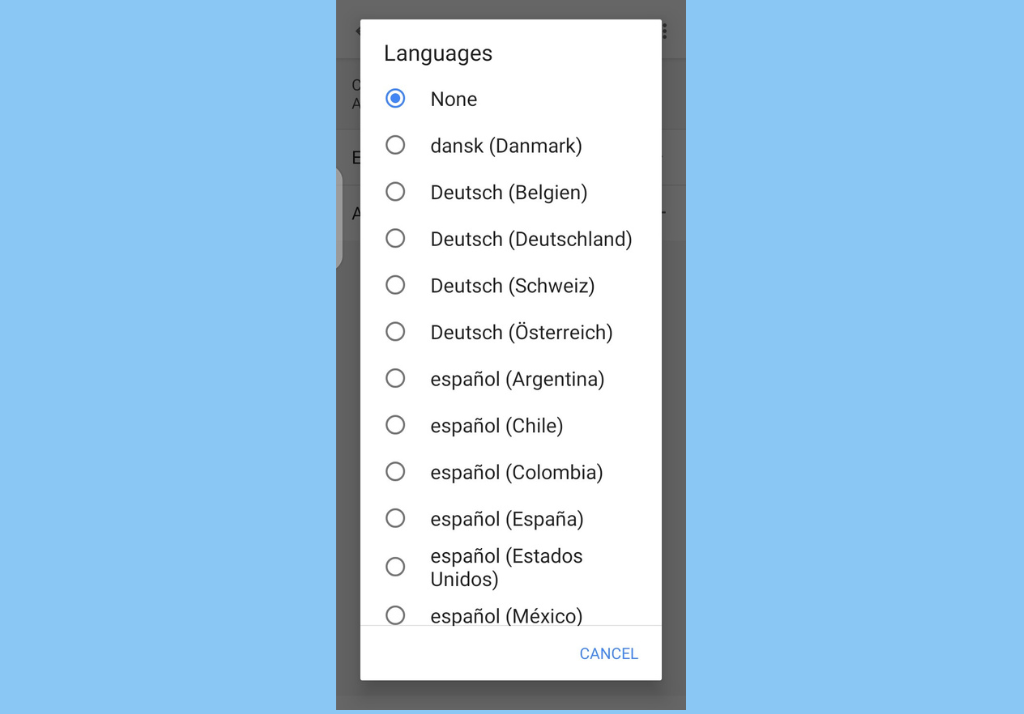The image features a predominantly blue background on the right and left sides, with a white rectangular section centered in the middle. The rectangle is outlined with a thick black border on all sides. At the top of the white section, the heading "Languages" is displayed.

Below the heading, there is a list of languages, each preceded by a circle, which suggests a selection option. The entries are left-aligned and include the following:

- None (selected with a blue fill in the circle)
- Dansk (Danish)
- Deutsch (German) 
  - Deutsch (Deutschland) 
  - Deutsch (Schweiz) 
  - Deutsch (Österreich)
- Español (Spanish) 
  - Español (Argentina) 
  - Español (Chile) 
  - Español (Colombia) 
  - Español (España) 
  - Español (Estados Unidos) 
  - Español (México)

At the bottom right corner, there is a button labeled "Cancel" in blue. The current selection in the list is "None", indicated by the blue fill in its corresponding circle. The list includes Danish, various forms of German spoken in Germany, Switzerland, and Austria, as well as several regional variations of Spanish.

The image likely represents a language selection interface, offering users the ability to choose their preferred language for an application or website.